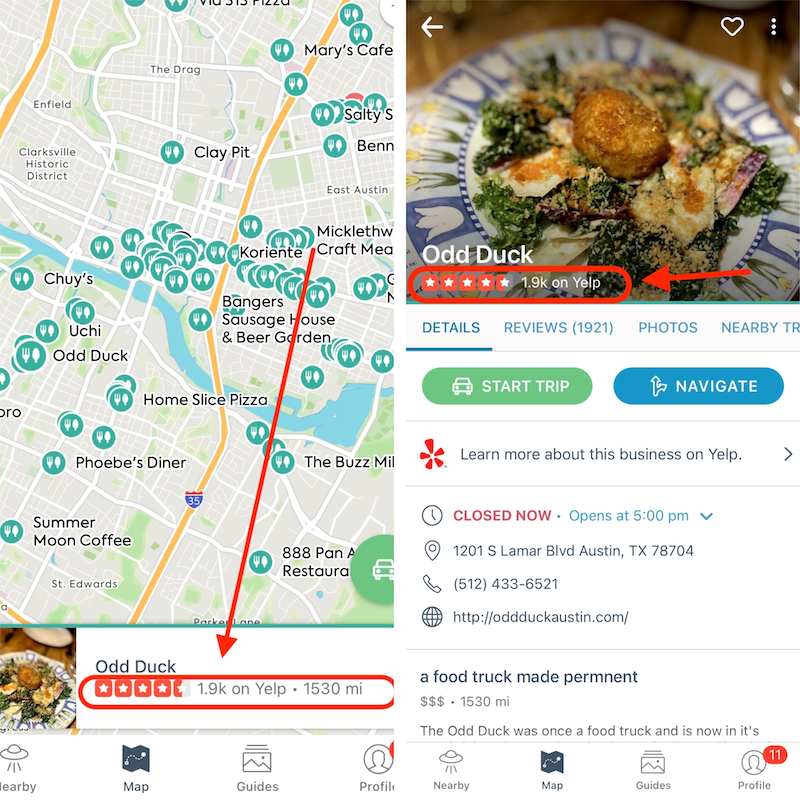The left side of the image prominently features a detailed map with various identifiers. White lines delineate different streets, while long orange lines segment distinct areas. The map is scattered with numerous small green circles marked with a fork and spoon icon, indicating places to eat. These eating spots are densely clustered, especially in the central area of the map. Some notable eateries include Banger's Sausage House and Beer Garden, Home Slice Pizza, Summer Moon Coffee, and Mickle Craft. A red arrow extends from the left side of the map, pointing to the bottom where "Odd Duck" is highlighted with a red circle. Odd Duck boasts a rating of 4.5 out of 5 stars, based on 1.9K Yelp reviews, and it is noted to be 1,530 miles away.

On the right side of the image, there is a plate of food featuring vegetables, eggs, and a fried item in the center. The dish is labeled "Odd Duck," accompanied by the same 4.5-star rating, corroborated by a red arrow pointing towards it. Below this, there is a section labeled "Details," underlined in blue, and a green, horizontal, oval button that reads "Start Trip." Next to this is a "Navigate" option.